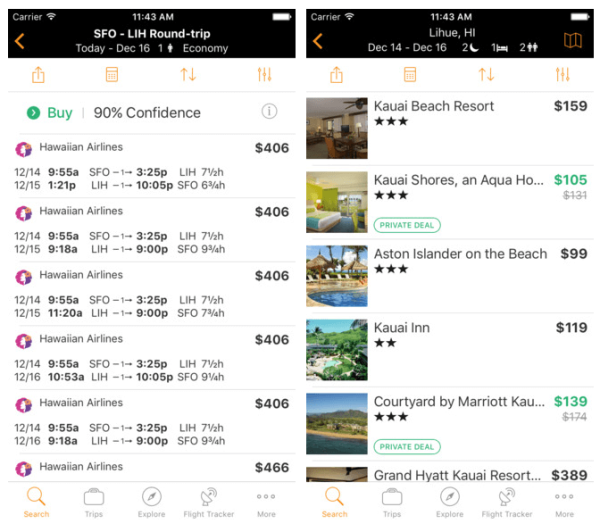The image showcases two different screenshots, likely from a smartphone due to the screen size, logos, and notifications. Both screenshots have a fully active Wi-Fi signal and display the time as 11:43 AM in the top center. The device's black bezel frames the screen.

**Left Screenshot Description:**
- **Header:**
  - Displays "SFO-LIH round trip" in bold white text.
  - Shows "carrier" at the top next to a full Wi-Fi signal icon.
  - Contains orange arrow indicators and date labels reading "today - December 16th."
  - Notes one traveler in economy class with "1 person" and an economy icon.
- **Navigation and Information Icons:**
  - Four icons for sharing, calendar, filtering, and advanced filtering.
  - Features a green circle with an arrow labeled "Buy" next to "90% confidence" in black text.
  - An information icon represented by a circle with an 'i'.
- **Flight Listings:**
  - Lists prices for round trips with Hawaiian Airlines, mentioning $406 as the fare.
  
**Right Screenshot Description:**
- **Header:**
  - States "LIHUE, HI, Luau, Hawaii" in bold white text.
  - Shows "carrier" at the top next to a full Wi-Fi signal icon.
  - Features orange arrow indicators and date labels "December 14th to December 16th," indicating a stay of two nights.
  - Specifies two people, with respective icons depicting two people and a bed for one night.
  - Includes an orange icon resembling a folded piece of paper.
- **Navigation and Information Icons:**
  - Four icons for sharing, calendar, filtering, and advanced filtering.
- **Hotel Listings:**
  - Lists various hotels and their prices:
    - KAUAI Beach Resort: $159.
    - Kauai Shores on Aqua (partially cut off): was $131, now $105 in green text.
    - ASTON Islander on the Beach: $99.
    - KAUAI Inn (2 stars): $119.
    - Courtyard by Marriott (partially cut off): was $174, now $139 in green text.
  - Each hotel has a star rating, with the number of stars varying between two and three.
- **Additional Details:**
  - A green "private deal" button on the lower left.